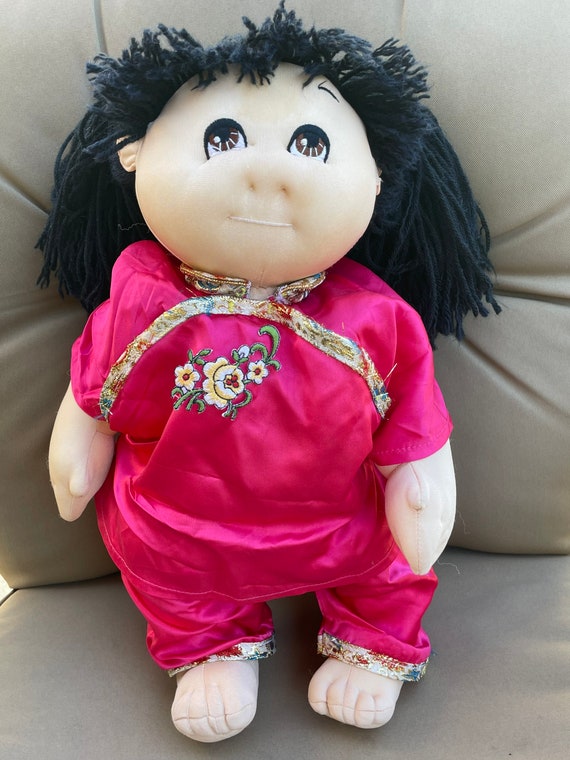The image depicts a handmade doll with dark black hair made of yarn or wool, styled to appear as if it's wearing traditional silk Chinese clothing. The doll is dressed in a bright pink satin outfit, consisting of both a top and pants, adorned with a vibrant floral pattern that includes colors like green, yellow, and white. The top of the outfit has floral designs across the chest and a shiny, possibly sequined trim both around the chest area and at the bottom of the pant legs. The doll's facial features include large brown eyes gazing upward, a small nose, and a straight line for a mouth, giving it a serene expression. It is displayed properly sitting on what appears to be a sofa or chair, enhancing its ornamental presentation.